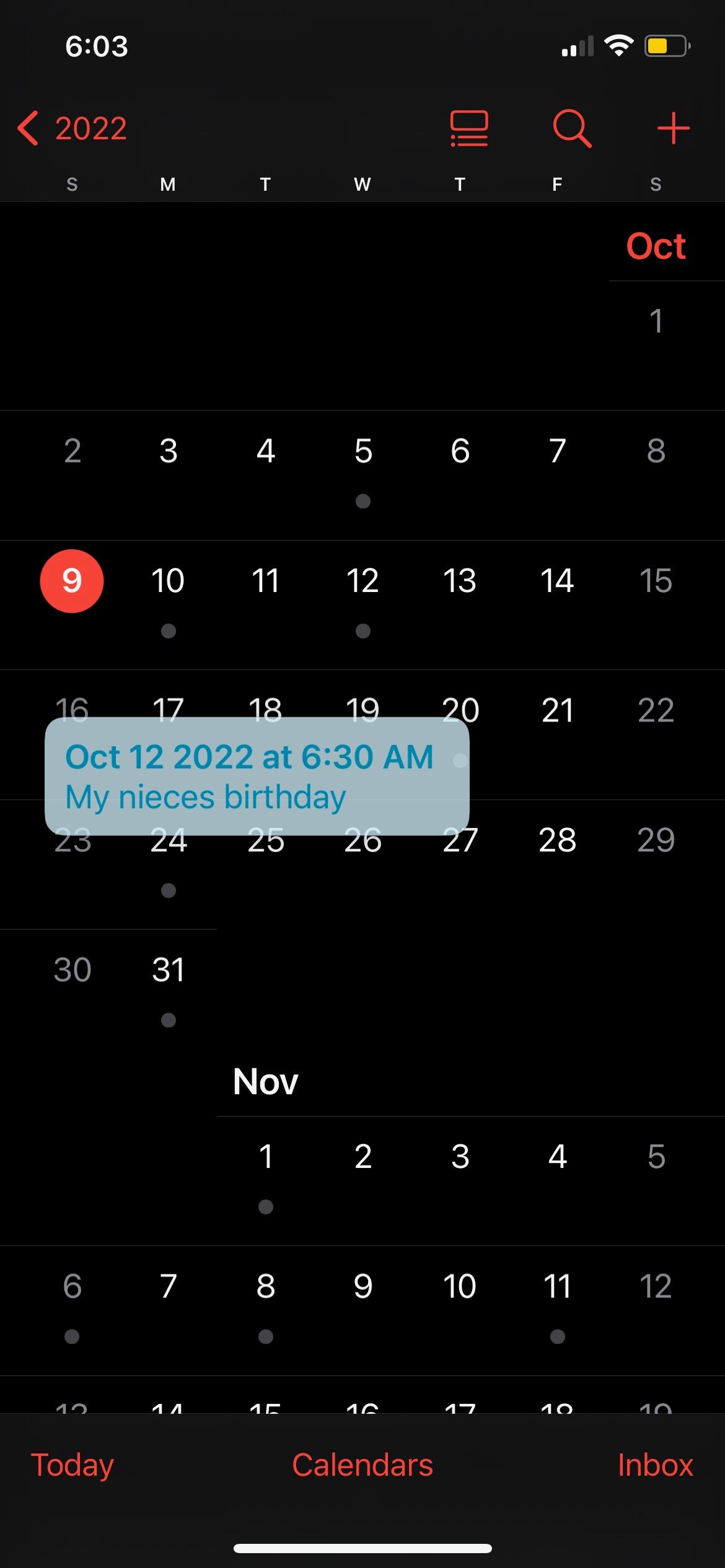In this screenshot, the time displayed on a solid black background is 6:03, as shown by the white text in the upper left corner. The upper right corner indicates the device's reception with two out of four bars lit up, Wi-Fi enabled, and the battery icon visible. The main focus of the image is an open calendar page for October 2022.

In the upper left part of the calendar, the year "2022" is seen above the month of October. To the right of this year indicator, there's a red magnifying glass icon followed by a plus sign. Below these icons, a row of days of the week is listed in white text, while to the far right, the word "October" is displayed in red.

A highlighted light gray box with blue text sits above the month of October, drawing attention to the specific dates within the month. A red circle emphasizes the date "9," indicating an event scheduled for that day. Further details within the highlighted box reveal the event details: "October 12th, 2022 at 6:30 a.m. - My niece's birthday."